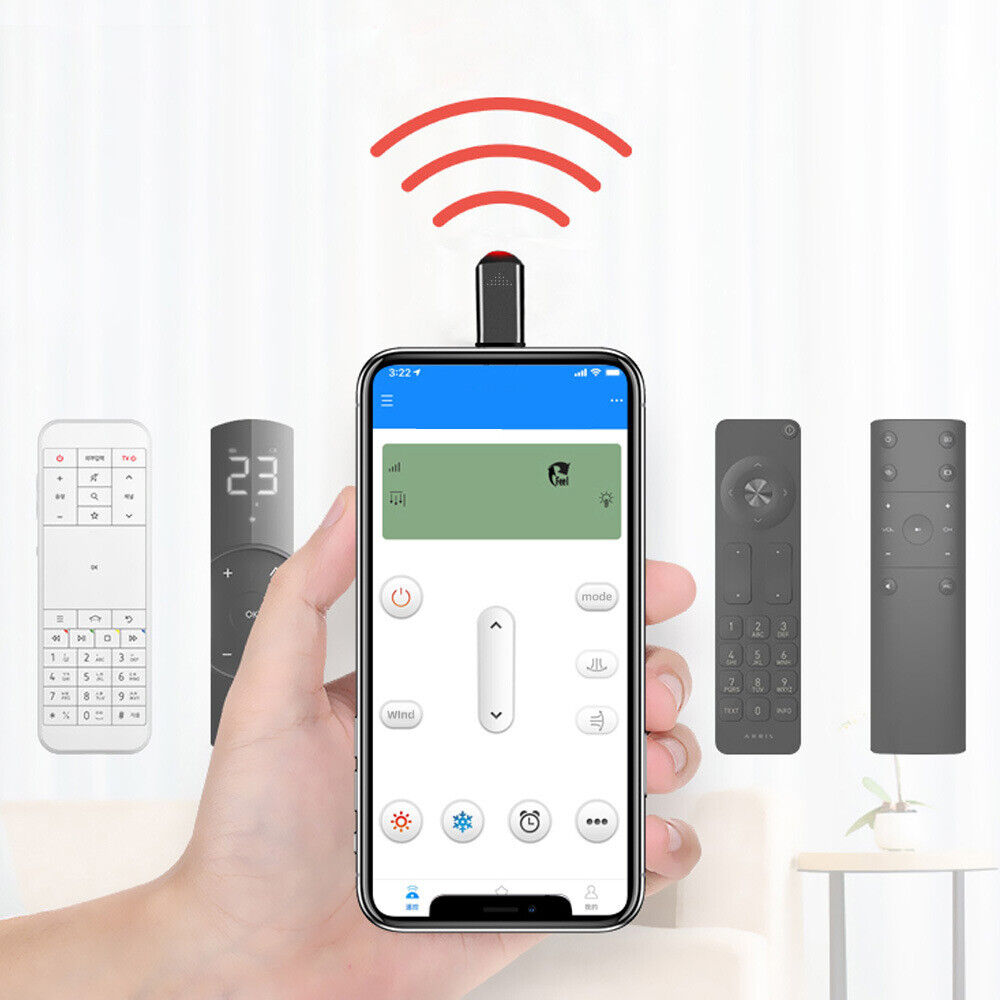The image depicts a hand grasping a cell phone with a small black device plugged into its top, emitting red lines suggestive of a wireless signal. The phone's screen displays various icons, including symbols for hot, cold, a timer, and an ellipse indicating additional options. In the background, there are several remote controllers: a white remote with square buttons, a black remote displaying "23" with plus and minus buttons, another black remote with square buttons and a round disc at the top, and an additional black remote with small round buttons. The setting also includes a small table adorned with a white bowl or vase containing a plant. This scene likely illustrates a system that integrates home heating control via a smartphone app connected to Wi-Fi.